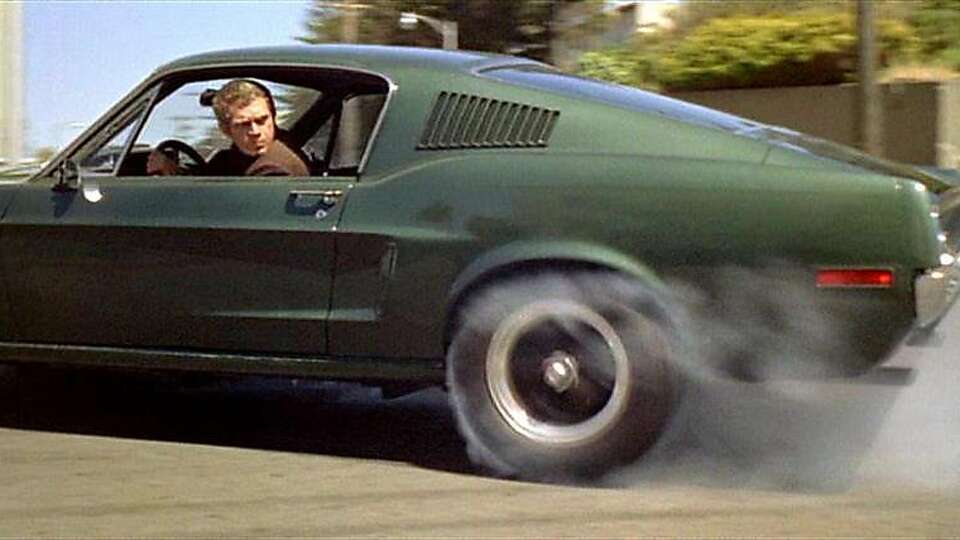The image captures a scene reminiscent of an old TV show or movie still, featuring a dark green muscle car, likely an old Mustang, possibly driven by someone resembling Steve McQueen. The sporty two-door vehicle is in motion, peeling out with smoke billowing from its back tires. The car is detailed with a distinctive grill on the side, black and white tires, and an indent that hints at its Mustang heritage. The driver, a white male with short blonde or brown hair, is wearing a brown jacket and is seen looking out his open window towards the back. The background reveals a plain wall topped with bushes and a streetlight, evoking an era gone by.